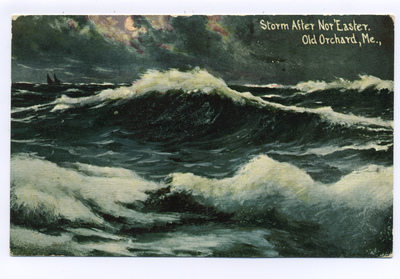This is an aged, postcard-sized painting with rounded and faded edges, capturing a stormy ocean scene. Dark grays, blues, and blacks dominate the tempestuous waves that are tipped with frothy white, conveying a sense of intensity and somberness. Above the ocean, the sky is midnight-dark with overcast clouds, lending to the painting's mysterious and foreboding atmosphere. A moon peeks through in the left-hand side, partially obscured by the clouds, while the silhouettes of two sailboats appear faintly in the distance with indistinct details. The top right corner features an off-white handwritten inscription that reads, "Storm after Nor'easter, Old Orchard, ME," indicating a connection to the northeastern United States.